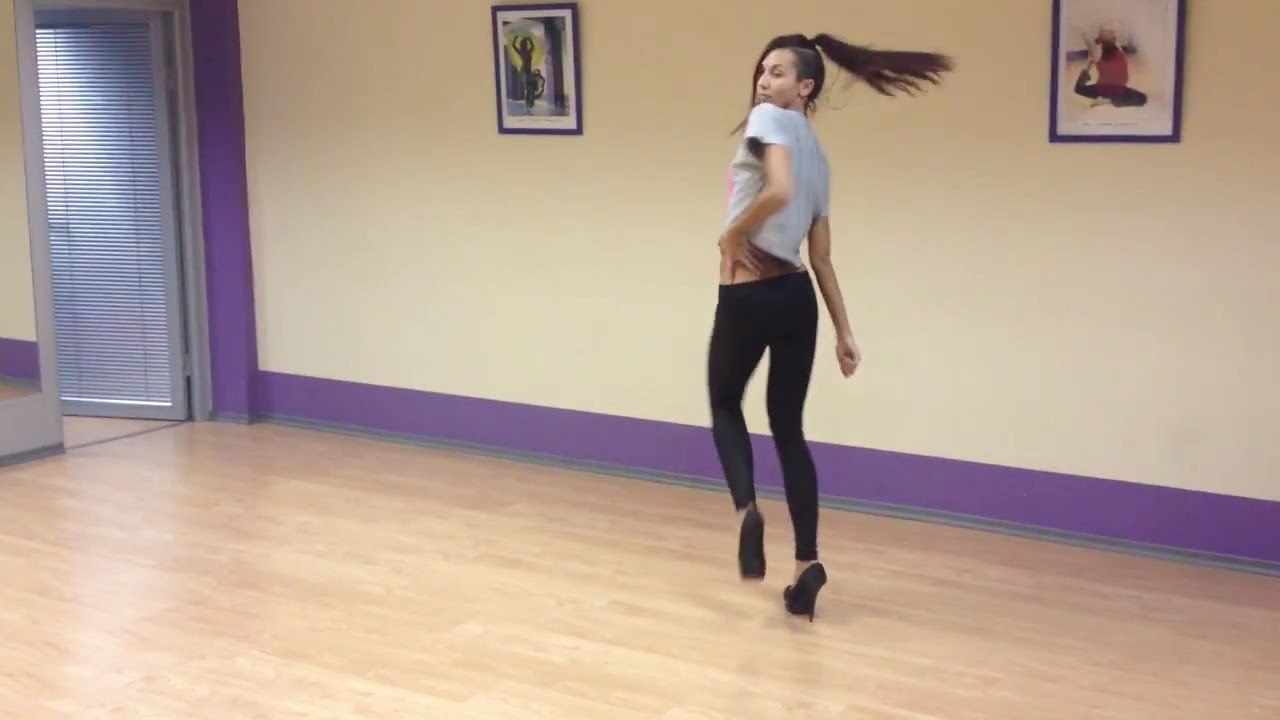In the image, a young, slender woman is captured mid-dance in a studio with light tan walls and a distinctive purple stripe running along the bottom edge. She dances gracefully on a light-colored hardwood floor, wearing black high heels—a challenging feat that she manages with impressive balance and poise. Her outfit consists of a gray t-shirt and tight black legging-like pants. Her long ponytail swings around, indicating her fluid movements, and she appears to be in motion, adding a dynamic, slightly blurry effect to the photograph. Her pose is striking, with her left hand placed confidently on her hip while she looks off to the side, seemingly towards a mirror to evaluate her dance moves. The dance studio is adorned with two large, framed posters spaced apart on the wall—one depicting a person stretching and the other showing someone dancing, enhancing the artistic ambiance of the space.